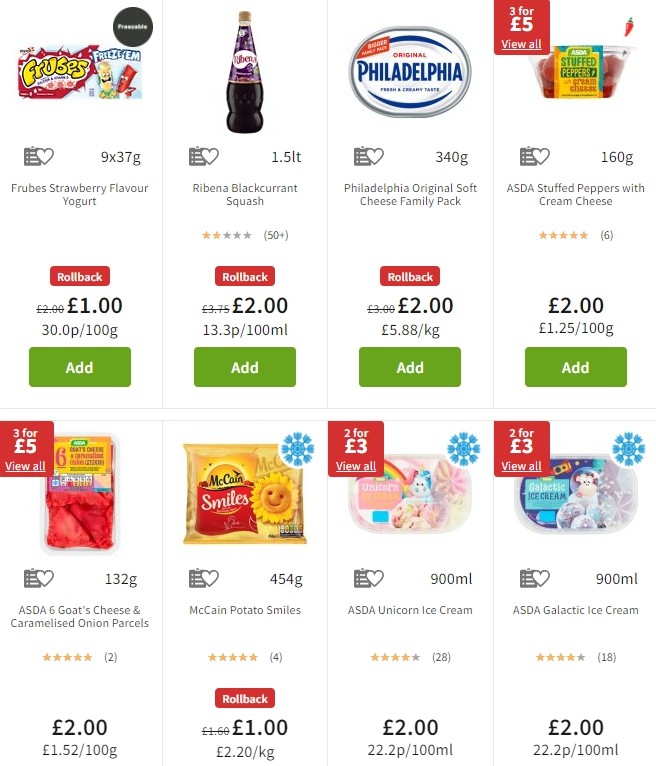The image displays a variety of grocery items with detailed information on prices, ratings, and promotional offers. Here is a detailed description of each item featured:

1. **Frubes Strawberry Flavor Yogurt**
   - **Brand**: Fruises/Freesome
   - **Price**: $1 (Rollback)
   - **Additional Information**: There is a green "add" button for easy purchase.

2. **Robina Blackcurrant Squash**
   - **Rating**: 2 stars out of over 50 ratings
   - **Price**: $2 (Rollback)
   - **Additional Information**: Green "add" button available.

3. **Philadelphia Original Soft Cream Cheese Family Pack**
   - **Price**: $2 (Rollback)
   - **Additional Information**: Includes a green "add" button.

4. **ASDA Stuffed Peppers with Cream Cheese**
   - **Price**: $2
   - **Promotion**: Part of a "Three for Five" deal.
   - **Additional Information**: Green "add" button and a "View All" option for more deals.

5. **ASDA Six Goat Cheese and Caramelized Onion Parcels**
   - **Price**: $2 each or part of the "Three for Five" deal.
   - **Additional Information**: Includes a green "add" button.

6. **McCain Potato Smiles**
   - **Rating**: 4 stars
   - **Price**: $1 (Rollback)
   - **Additional Information**: Green "add" button available.

7. **ASDA Unicorn Ice Cream**
   - **Price**: $2 each or two for $3.
   - **Additional Information**: Includes a green "add" button.

8. **ASDA Galactic Ice Cream**
   - **Price**: $2
   - **Additional Information**: Contains a green "add" button for convenience.

The detailed promotional offers and ratings provide valuable information for customers looking to make an informed shopping choice, and the green "add" buttons facilitate quick and easy addition to their shopping cart.